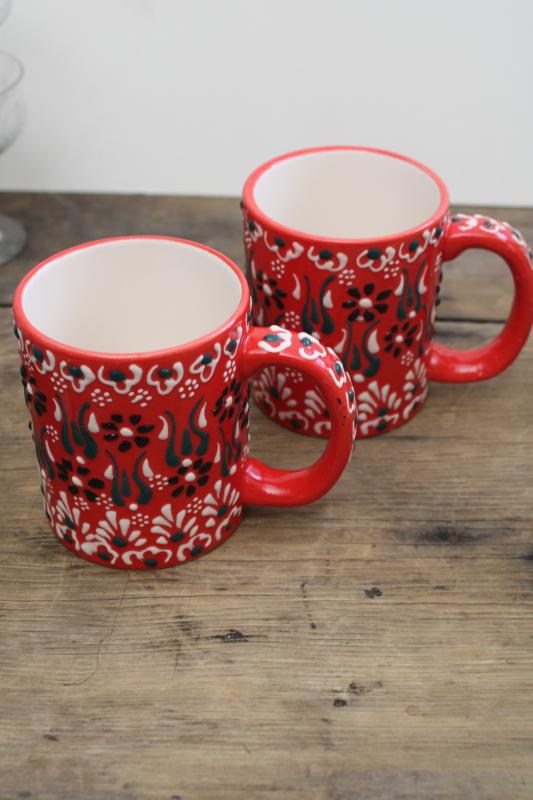This color photograph captures two identical coffee mugs sitting on a distressed brown and black wooden surface. Both mugs are white on the inside and have an elaborate red exterior adorned with a variety of black and white floral and geometric patterns. The mugs feature red handles with intricate white and green decorations, all facing to the right. The upper rims are encircled with patterns of dots and semicircles that resemble floral designs, while the midsections have black flower petals with white central dots and adjacent squiggly lines reminiscent of seaweed. The bottom sections are adorned with teardrop-shaped white petals and black dots. Behind the mugs, the background wall is white, and at the upper left corner of the image, part of what appears to be a clear glass vase is visible. The mugs are empty, emphasizing the detailed artistry on their surfaces.